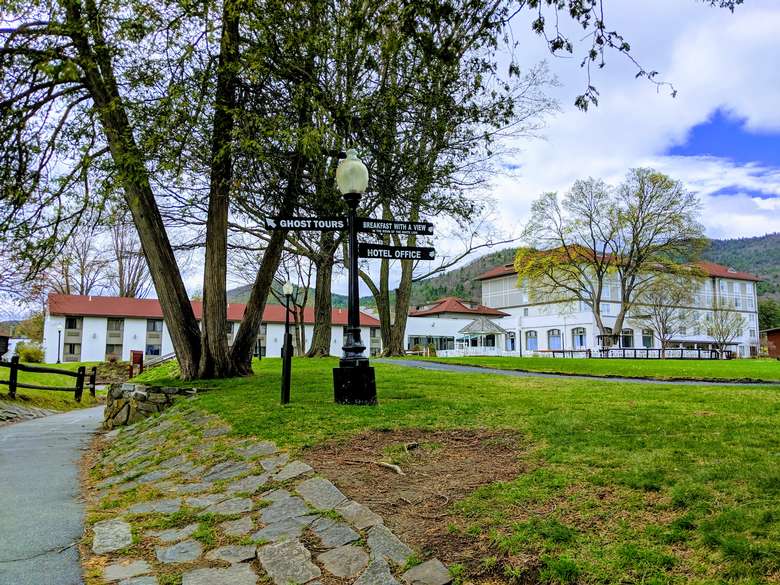The image features a picturesque scene with two prominent white buildings, each topped with a red roof, set against a scenic backdrop of tree-covered hills and a partly cloudy sky. The building on the left is two stories tall, whereas the building on the right stands taller, approximately five stories high, and both structures appear to be disconnected yet similarly styled. In the foreground, there's a small grassy area intersected by a horizontal asphalt pathway. On the left side of the image, another pathway leads towards the left building, flanked by a small berm of flat stones and a short lamppost bearing signs. These black signs with white text indicate directions for "Ghost Tours," which points to the left, and "Hotel Office" and "Breakfast with a View," both pointing to the right. A few trees are scattered around the grassy areas near the lamppost. The scene exudes calmness with its manicured landscape and the distant, rolling hills that add a sense of depth and tranquility to the setting, suggesting a charming, possibly historic, hotel or plantation house in a tropical or temperate locale.